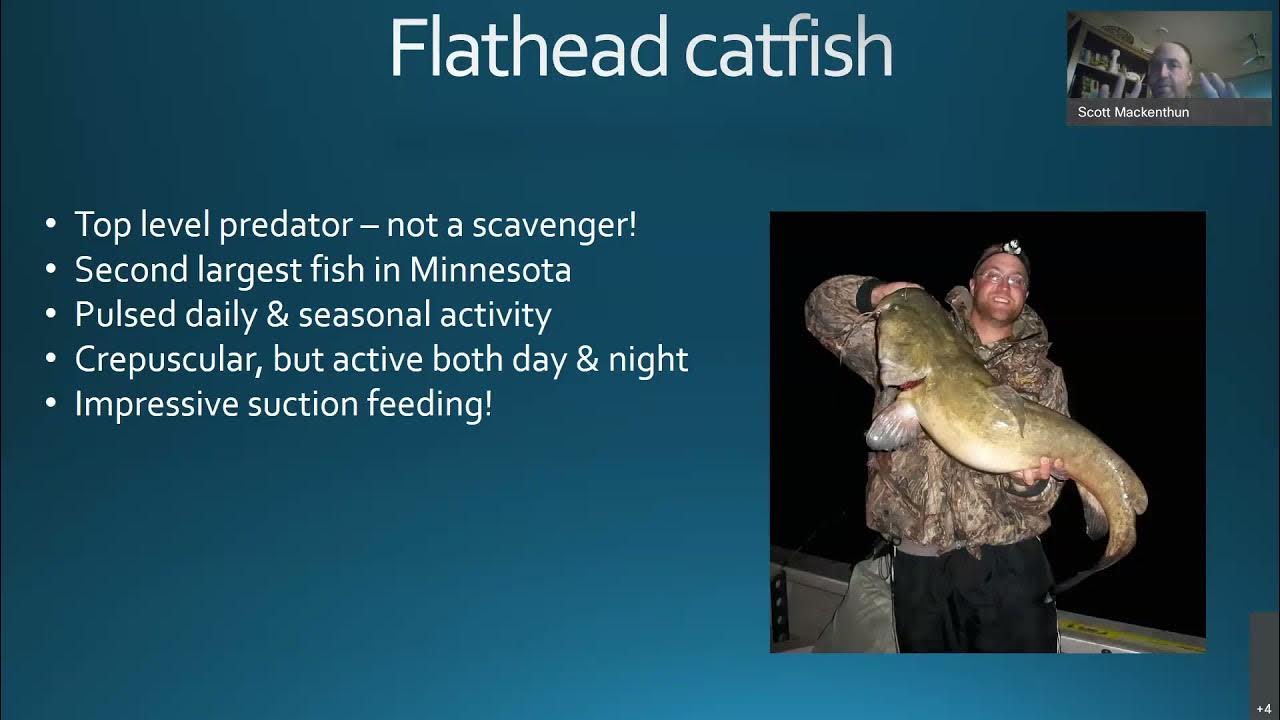The image is a slide from a presentation with a blue background and white font, titled "Flathead Catfish" at the top. The slide features five bullet points on the left side that describe the fish as follows: "Top-level predator, not a scavenger," "Second largest fish in Minnesota," "Post daily and seasonal activity," "Crepuscular but active both day and night," and "Impressive suction feeding." On the right side of the slide, there is a nighttime photograph of a man in a camo jacket and black pants, standing in a boat and holding a large, greenish-brown flathead catfish with hints of yellow. In the upper right corner of the slide, there appears to be a webcam image with the name "Scott Mackenthun" displayed, showing a person waving.